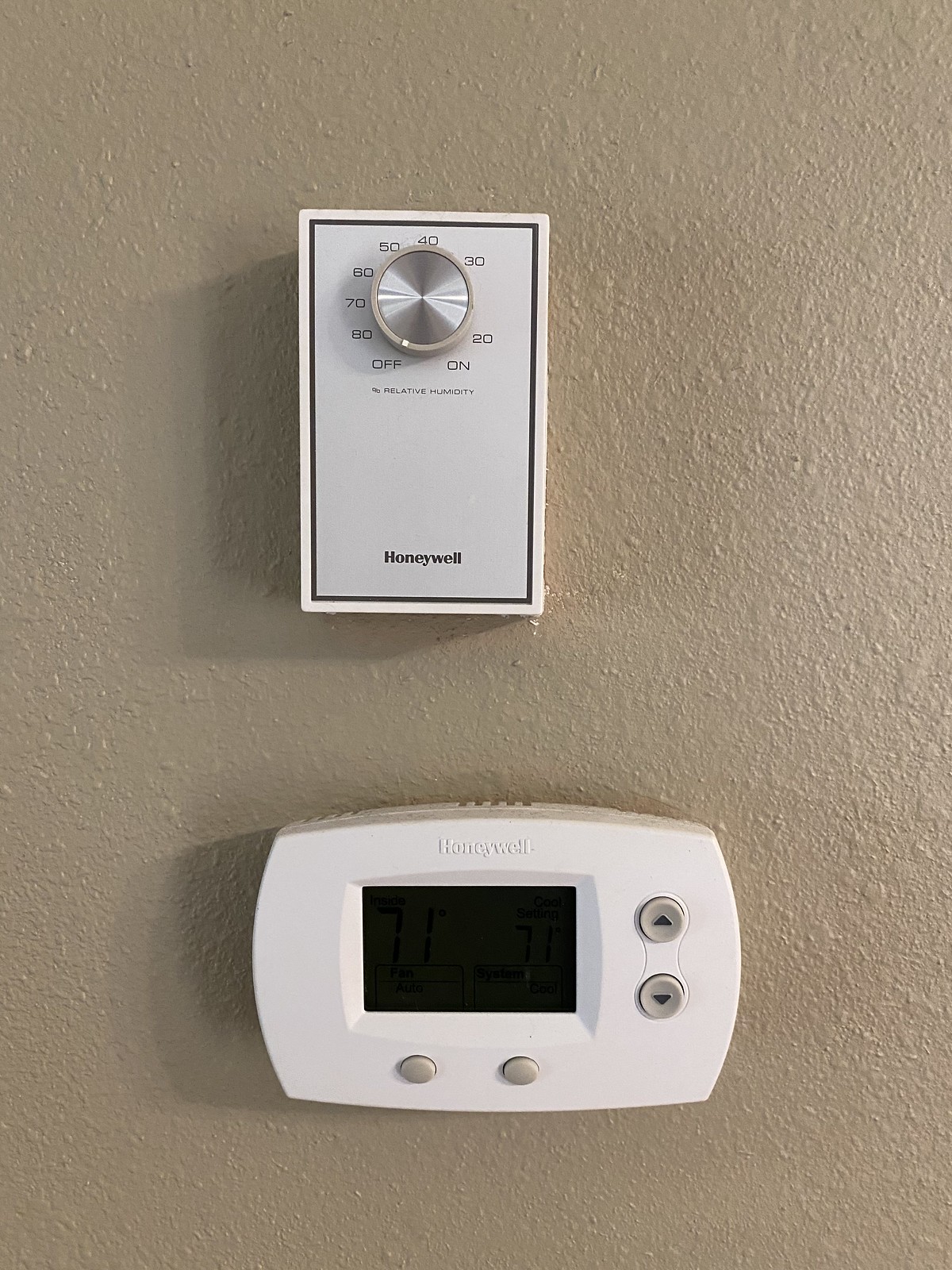The close-up photograph features two distinct home thermostats affixed to a popcorn-textured wall painted in a shade of taupe. 

The thermostat at the top presents a vintage design. It is a vertically oriented, rectangular device with a white casing and a silver faceplate, bordered by black. Central to its design is a circular dial, which is currently set to the “off” position. The dial itself is silver with a gray perimeter, housing a small white circle at its peak. The dial's temperature range is clearly marked in increments, displaying numbers 20, 30, 40, 60, 70, 80, and 90 degrees. Positioned on the lower right is the "on" designation, while the perimeter of the dial is inscribed with small, black numbering. At the base of this thermostat, the brand name "Honeywell" is subtly printed in small black letters.

Directly beneath the vintage model sits a more contemporary thermostat, centered in the photograph. Encased in white plastic, this device also bears the "Honeywell" brand, this time embossed in raised white lettering at the top. A black digital panel, centrally located, serves as the focal point of this modern thermostat. To its right are two tactile, gray buttons marked with black triangles for adjusting the temperature up and down. Additionally, it features another two gray buttons located on the left and right sides of the device's front panel.

The composition of the image creates a striking comparison between the old and new thermostat designs, both unified in their functionality yet distinct in their aesthetics.